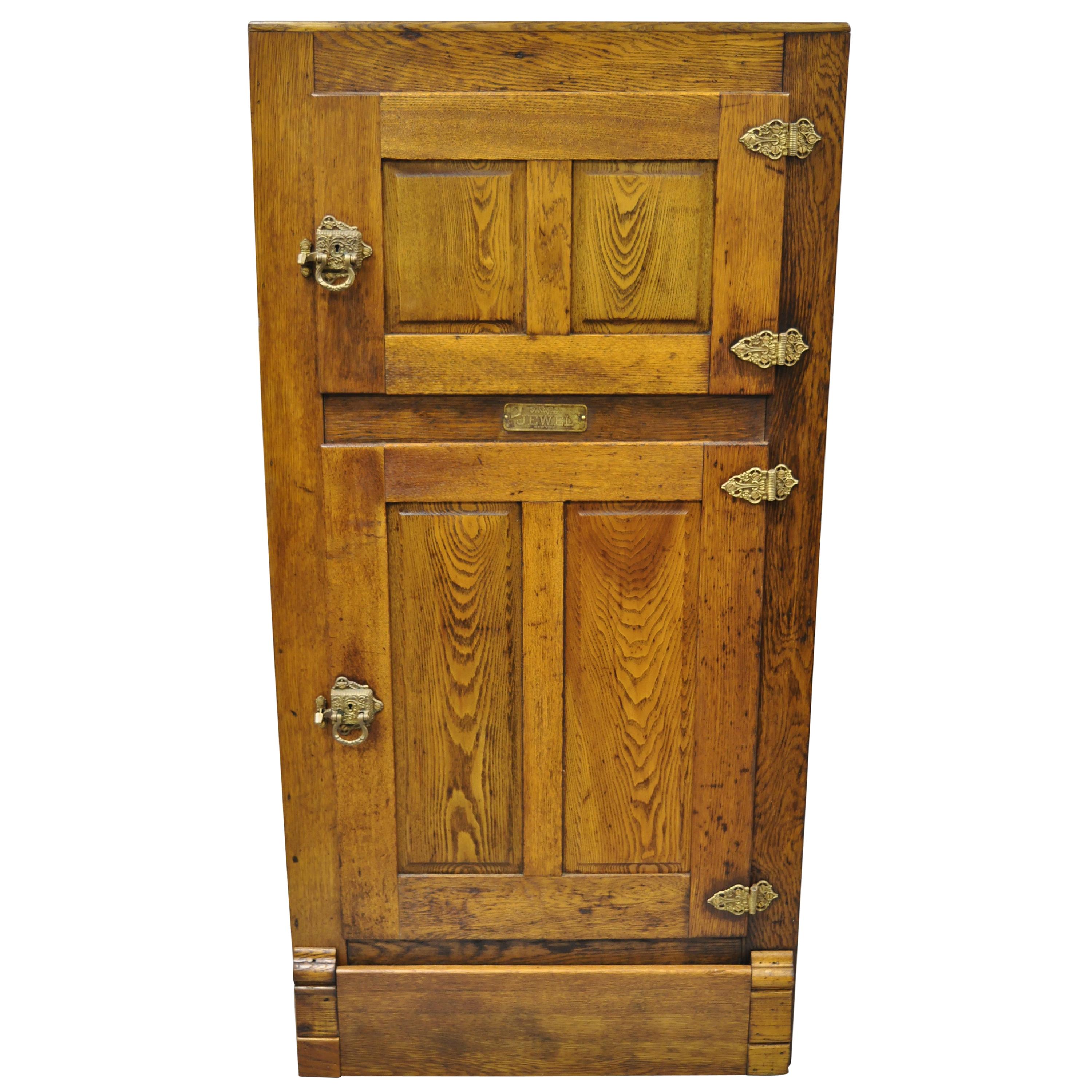The image showcases a beautifully crafted vintage oak icebox with two doors, one smaller upper door and a larger lower door. Both doors are constructed of finely grained oak wood, with each door featuring two rectangular panels. The wood is stunning in its natural details, highlighted by the characteristic patterns and grains of oak. Ornate brass hinges and matching heavy brass latches adorn the doors, reflecting an era of meticulous craftsmanship. Between the two doors, a metal identification plate is affixed, although the text is not legible. The doors are accessorized with intricate handles that operate the locks, allowing them to slide for securing each door. While the overall design is simple, with no carvings, the paneling and the brass details bring out the elegant, functional beauty of this well-preserved piece.